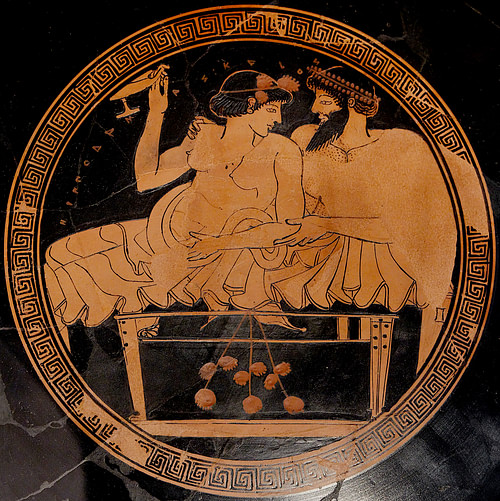This image depicts an ancient Greek or Roman-style plate against a shiny, black marble-like background. The round plate has a circular, helical patterned border with a worn appearance, suggesting its age. The central image is crafted in black and a golden-orange hue. It portrays a man and a woman, both topless and adorned in Roman-like drapery from the waist down. The man, situated on the right, has a long black beard and wears a laurel wreath. The woman, on the left, has reddish flowers in her hair and holds an Aladdin's lamp in her right hand, lifted above her head. They are seated on a rectangular structure decorated with flowers. The scene exudes a peaceful, harmonious vibe as the couple looks fondly at each other.